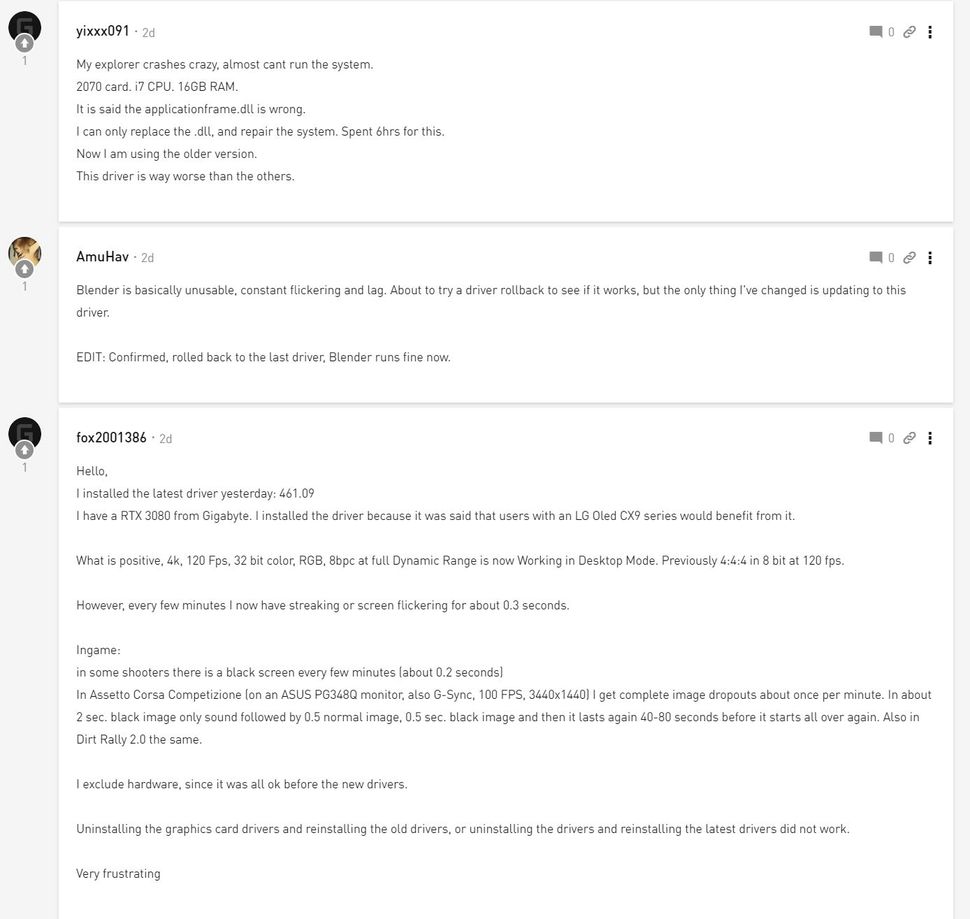Screenshot of an online discussion featuring three users, each sharing their disheartening experiences with their system performance after installing a new graphics driver:

1. **YIXX091** - 2 days ago: "My Explorer crashes constantly, making the system nearly unusable. I have a 2070 GPU, i7 CPU, and 16GB RAM. An error with the application frame DLL forced me to spend 6 hours replacing the DLL and repairing the system. Now, I'm using an older driver version, which performs worse than the others."
  
2. **AMUHAV** - 2 days ago: "Blender has become basically unusable with severe flickering and lag. I'm planning to roll back the driver update to see if it solves the issue. Edit: Confirmed, the rollback to the previous driver fixed Blender's performance."

3. **FOX2001-386** - 2 days ago: "I installed the latest driver (461.09) yesterday for my Gigabyte RTX 3080 to benefit my LG OLED CX9 series. Unfortunately, I now experience frequent streaking and screen flickering. In some shooter games, I encounter black screens every few minutes. I'm uninstalling the graphics card driver and reverting to the previous version out of frustration."

The conversation highlights the users' frustrations with recent driver updates causing significant system instability and performance issues, leading to their turning back to older, more stable versions.